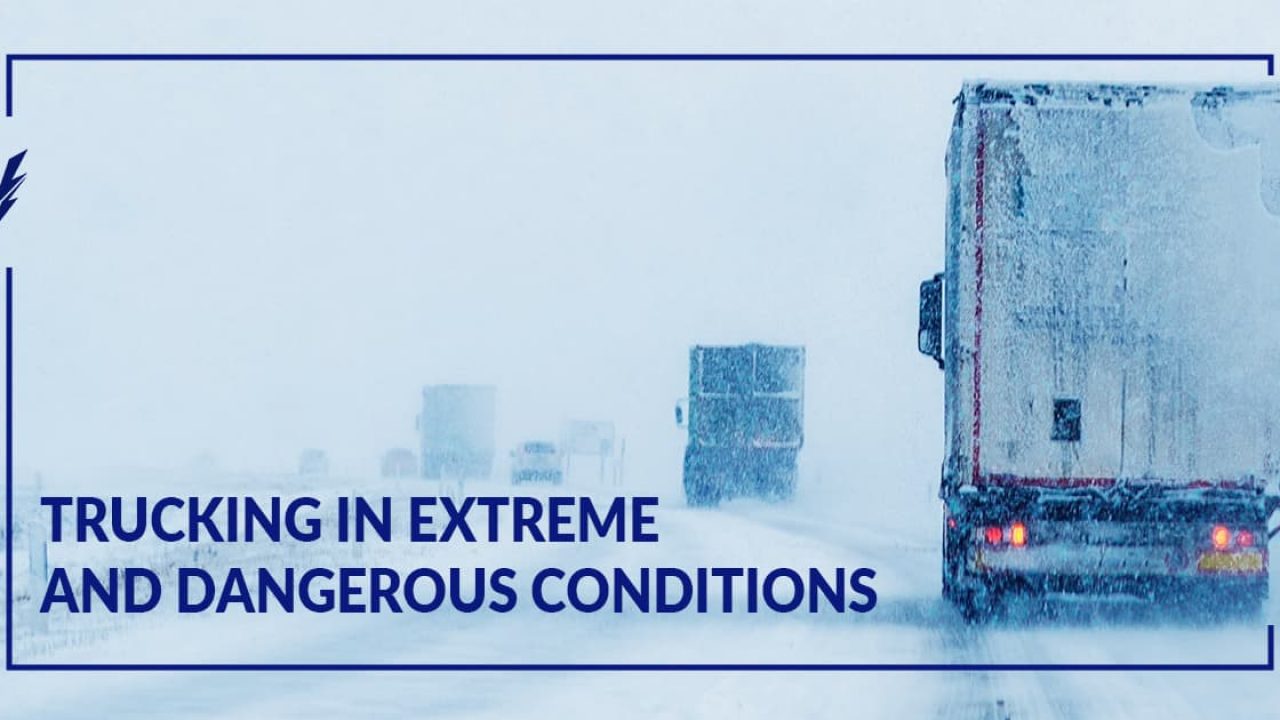The photograph is a horizontal rectangle capturing a treacherous winter scene on an icy highway during an extreme snow blizzard. Visibility is severely impaired due to the heavy snowfall and fierce wind, creating a whiteout effect. In the image, you can discern six trucks, each progressively fading into the snowy horizon. The closest truck, partially shrouded in ice, has its taillights illuminated, its cabin covered in a layer of frost, and tire tracks are visible in the snow. The photo, which might be the first slide of a PowerPoint presentation intended as a guide for driving in severe winter conditions, features blue text that reads "Trucking in extreme and dangerous conditions." Additionally, a blue border frames the image, adding a subtle yet continuous emphasis around the photograph.